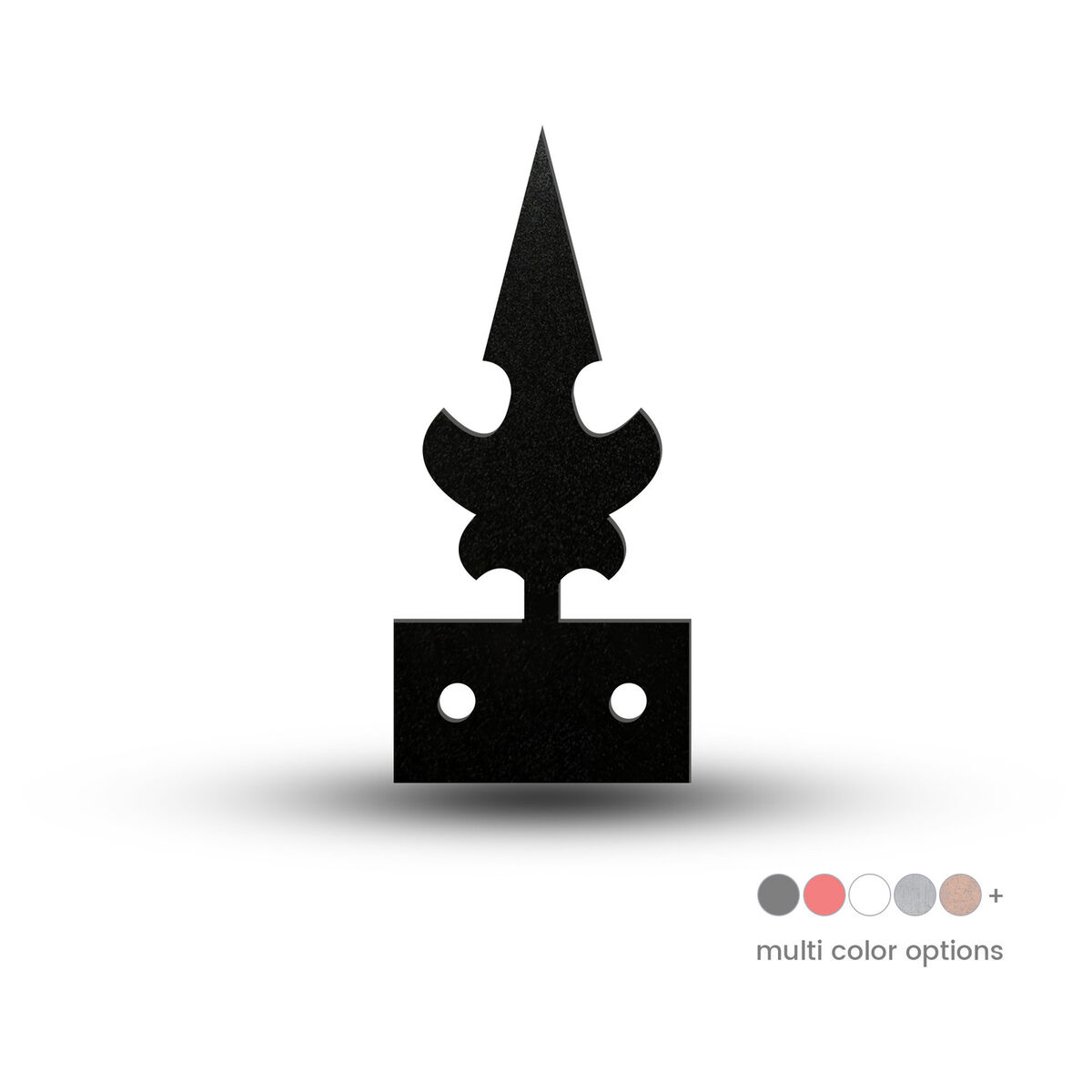This image showcases a black, metallic spear-like finial, commonly used on top of fences. The finial features a pointy spearhead design, followed by a leaf-like motif beneath it, both of which contribute to its decorative appearance. The intricate design sits atop a rectangular base with two round holes. Below the rectangular surface, a gray shadow is visible, indicating the three-dimensional aspect of the finial. In the bottom right corner of the image, there are several small circles in various colors—dark gray, pink, white, light gray, and beige—labeled "multi-color options." Additionally, a plus sign is positioned to the right of these circles. The background of the image is entirely white, providing a stark contrast that highlights the black finial and the colorful selection circles.